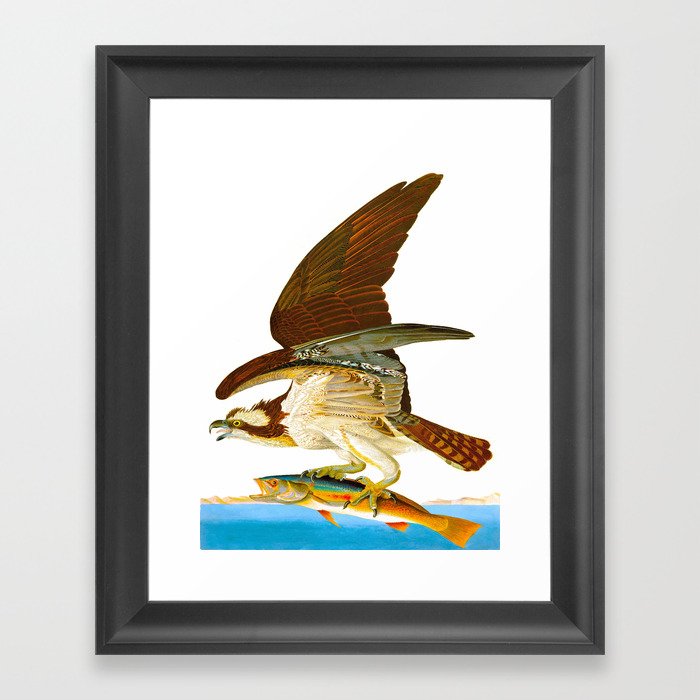In this detailed image, we see a black-framed photo with a portrait orientation hanging against a light gray background. The photo itself is set on a white mat, emphasizing the vivid scene it captures. The centerpiece is an eagle in flight, depicted with a realistic artistic style. The eagle has brown wings with intricate patterns and a white underbelly, complemented by a distinct head featuring brown and white feathers, an open beak, and visible tongue. It is portrayed in mid-action, lifting a large fish with its sharp talons from the vibrant blue water below. The water surface, along with a few brown mountain hills on the shore, forms the lower part of the composition. The fish, caught in the eagle's powerful grasp, is characterized by a blue back, an orange tail, and fins, with a white underside. Above the dramatic scene, the background transitions into a stark white sky, highlighting the eagle's powerful wings and the fine details of its feathers as it soars to the left. This photographic representation captures the dynamic interplay of nature's predator and prey, framed exquisitely to bring out both the action and the beauty of the moment.